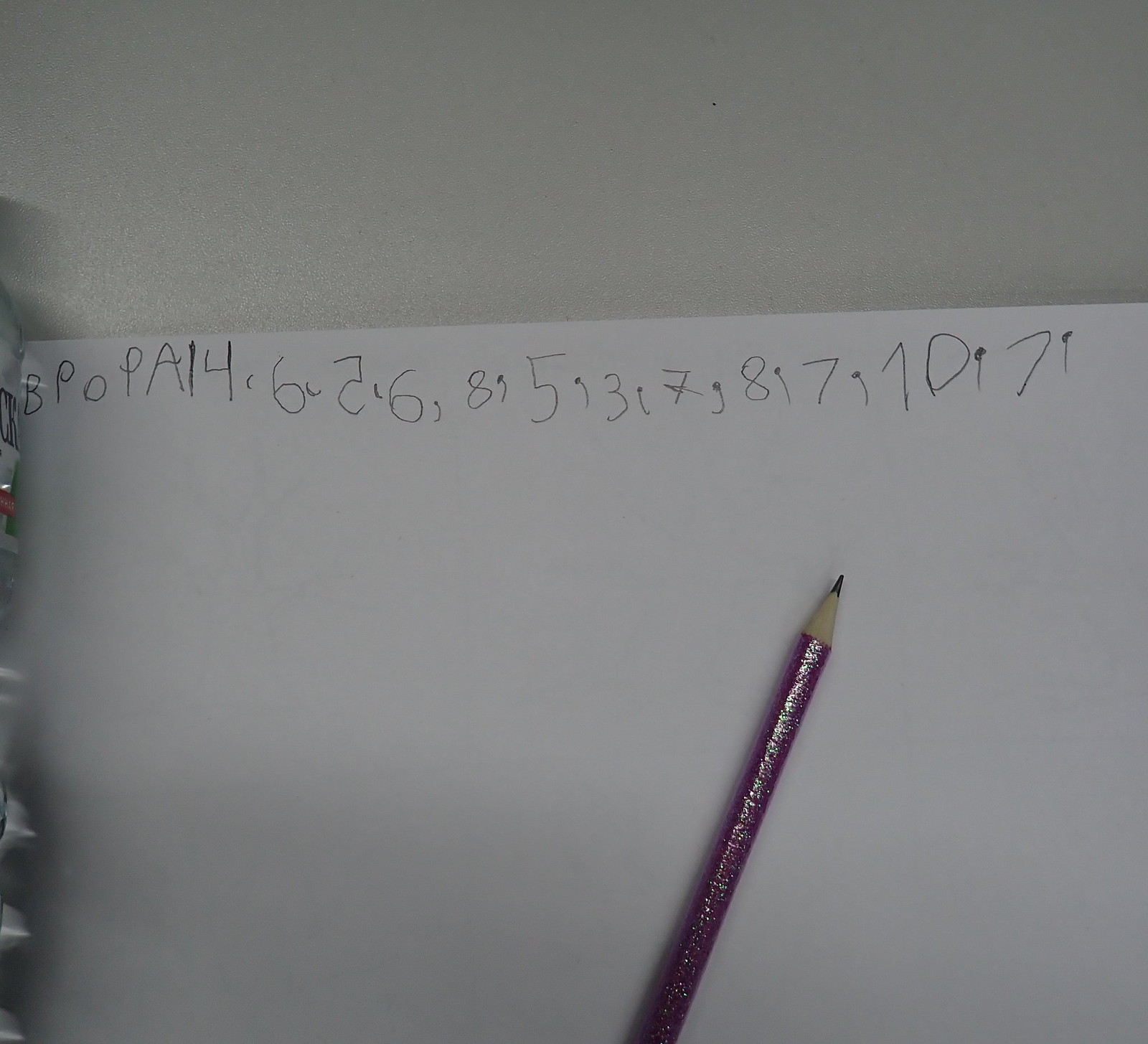In this detailed photograph, a sharpened pencil with a glittery silver handle and a purple shaft rests atop a piece of paper. The pencil appears freshly sharpened and ready for use. The paper, which is positioned on a table, features a mix of numbers and letters handwritten at the top in a seemingly random arrangement. The sequence includes: a capital 'B', a capital 'P', 'O', another capital 'P', 'A', followed by the numbers 1, 4, a backward 5, and a series of numbers separated by commas - 6, 8, 5, 3, 7, 8, 7, and 10. The overall scene suggests an impromptu note-taking or brainstorming session, with the vibrant, glittery pencil standing out as the focal point.